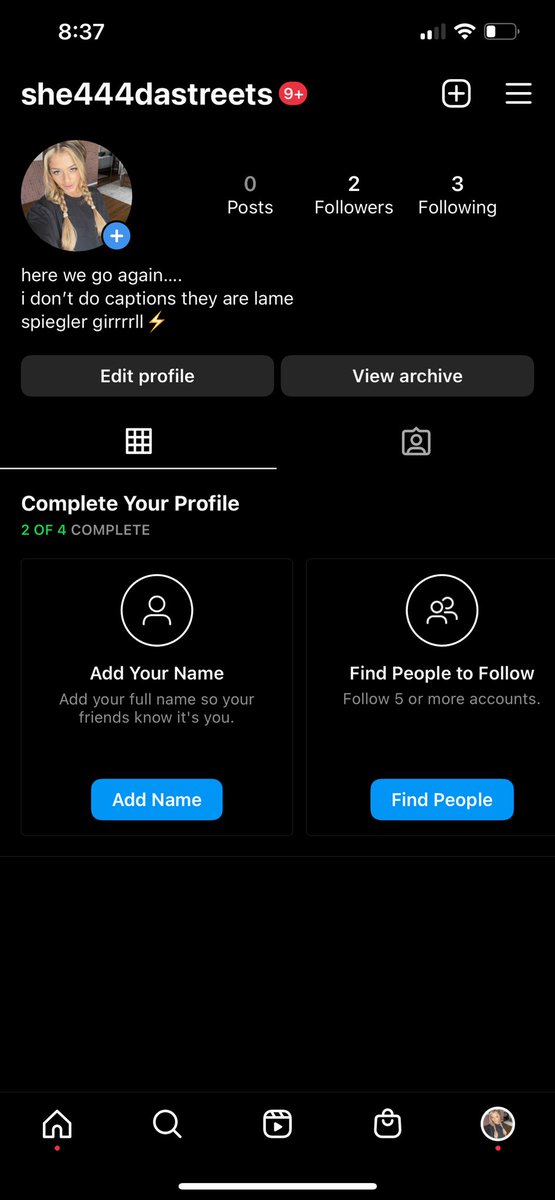In this screenshot taken on an iPhone, the distinctive layout and icons confirm the device type. At the top of the screen, the status bar indicates the Wi-Fi is enabled, the battery level is low, and the phone is not charging. The time displayed is 8:37, though it is unclear if it is AM or PM.

The screenshot captures an Instagram profile belonging to a user named "she44thestreets." This user has 2 followers and follows 3 accounts. The profile picture shows a white Caucasian girl with two pigtails. Her bio reads, "here we go again, I don't do captions." Additionally, there is a prompt to view her archive and a suggestion to complete her profile by adding a name and finding more people to follow.

At the bottom of the screen, the typical Instagram navigation bar is visible, featuring five icons: Home, Search, Reels (Play), Shopping (Store), and Profile.